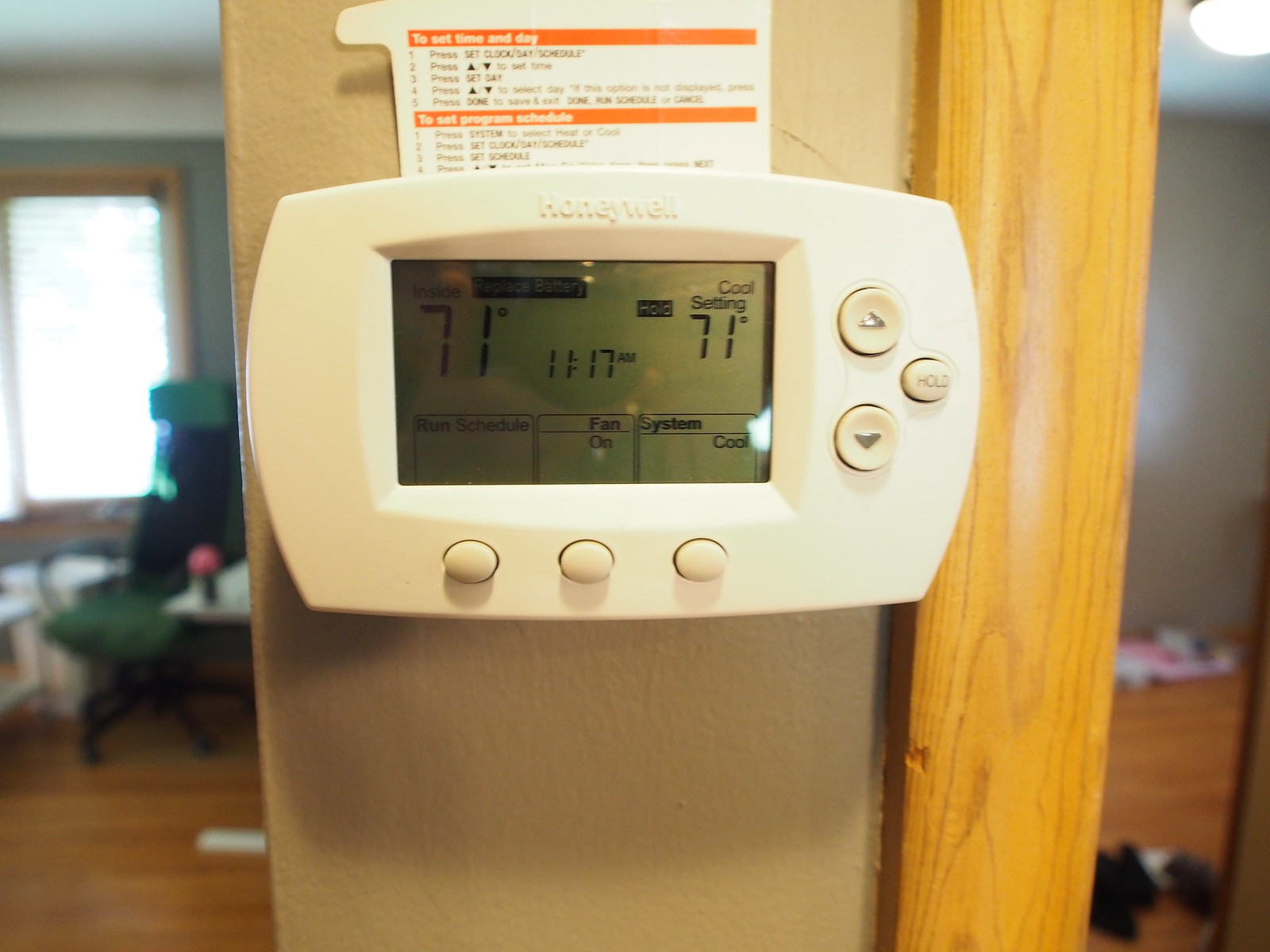This image features a white, somewhat bulky thermostat with a rectangular shape and curved edges. Located on the right side of the device are three buttons: one at the top, another below it, and a third positioned off to the side, midway between the two. The center of the thermostat showcases a screen displaying readings such as "71" and "11:17," alongside additional controls. The thermostat is mounted on a gray-beige wall. In the background, a cluttered room is visible with a person present, along with a chair and a nearby table strewn with items.